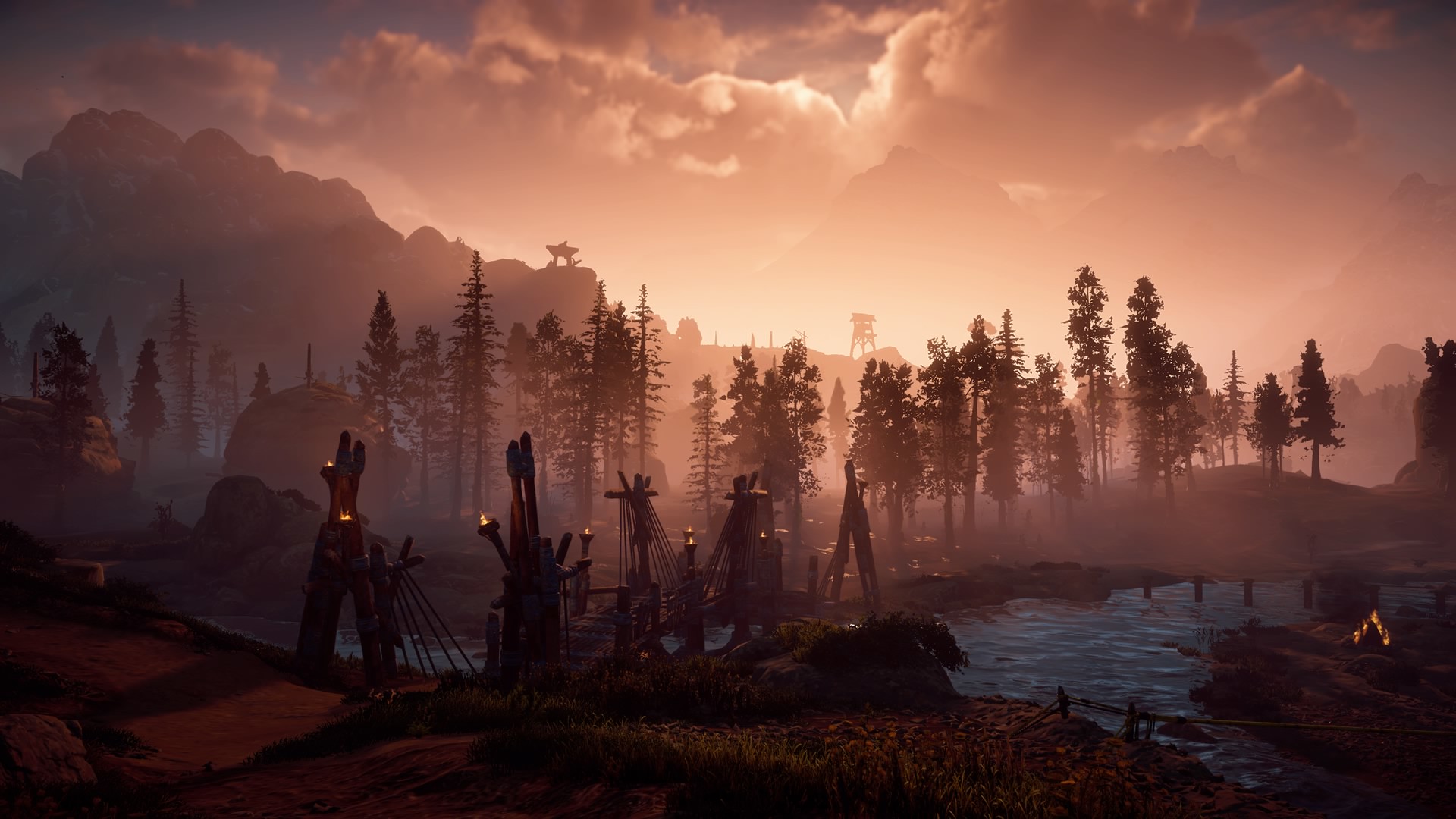In this detailed, computer-generated landscape illustration, we are set in a forest-like environment with jagged mountain ranges extending from left to right. The mountains, some of which sport objects like an antenna tower and a solitary tree, diminish in size from the leftmost, tallest peak to the smaller ones on the right. Above, the sky is heavily laden with thick clouds, most of which possess a pinkish hue, except for a central portion that remains white. Illuminating the scene is a gentle light filtering through these clouds.

In the foreground, a wooden, V-shaped bridge ornamented with ropes or cables and flaming torches stretches across a body of water that reflects a clear blue hue. The bridge, which seems to convey travelers from a rear landmass to the landmass at the bottom of the screen, is flanked by lush pine trees. Below the mountains, a sparse forest with dozens of tall, narrow trees adds more greenery to the scene, blending seamlessly with the grassy patches encircling the dirt trail visible at the front.

On the immediate right of the screen, separated yet visually integral, is another landmass that appears brown with an illuminated triangular object. Finally, the entire illustration, rendered in harmonious pink and brown hues, reveals scenic low-lying grass hills that slope down to the river, completing the picturesque and serene setting.